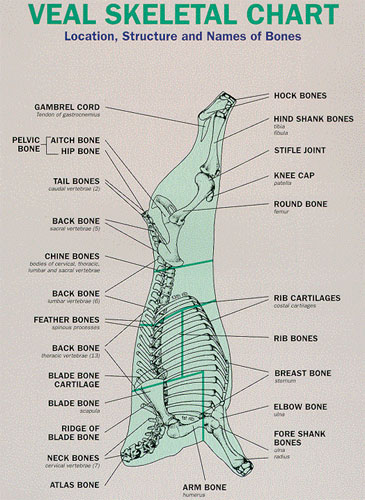The image is a detailed anatomical chart of a veal skeleton, resembling something you might find in a doctor's office. It is set against a light gray background and is labeled at the top in green lettering as "Veal Skeletal Chart" with the subtitle "Location, Structure, and Name of Bones." The veal is depicted hanging vertically without a head, exposing its skeletal structure. Various bones are meticulously labeled with lines pointing to each part. 

On the left-hand side, a vertical list identifies the gabriel cord, pelvic bone, ateach bone, hip bone, tail bones, backbone, chine bones, backbone (repeated), feather bones, backbone (repeated again), blade bone cartilage, blade bone, ridge of blade bone, neck bones, and atlas bone. On the right-hand side, labels delineate the hock bones, hind shank bones, stifle joint, kneecap, round bone, rib cartilages, rib bones, breast bone, elbow bone, fore shank bones, and arm bone. The chart provides a comprehensive look at the bone structure of the veal, showcasing both common and specialized terms for each part of the skeleton.